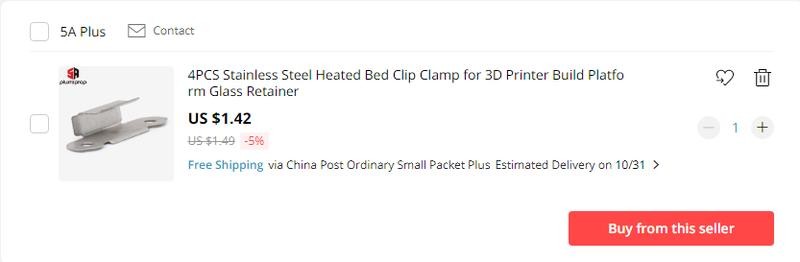The image appears to be a screenshot from an e-commerce website. The overall background is white. At the top, there is a light gray line running across the page. Below this line, in the top-left corner, is a gray-outlined box containing text and icons. The text, in black, reads "5A+". Adjacent to this text is an envelope icon followed by the word "CONTACT" in capital letters.

To the right of this section is a large white space. Directly beneath, there is another gray-outlined square. Inside this square, there is an image of a steel bed clip clamp. Next to the image is the detailed product description that reads: "4PCS stainless steel heated bed clip clamp for 3D printer. Built PLATFORM glass retainer." The price listed for this item is $1.42 USD.  

At the bottom-right corner of the image, there is a rectangular red background featuring the text "Buy from the seller" in white letters.